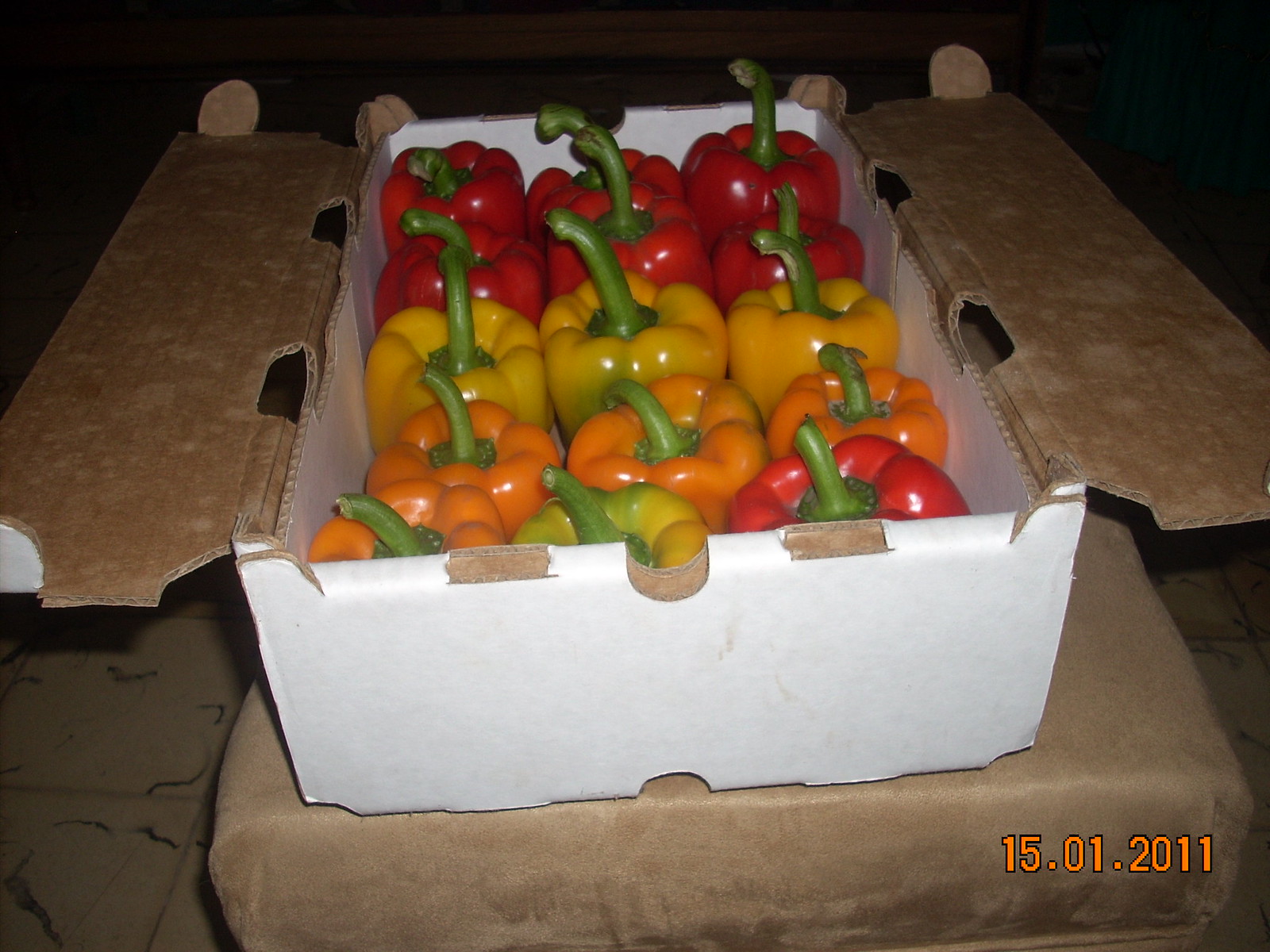This image, illuminated by camera flash in a dark room, captures a white cardboard box holding a neat arrangement of 15 bell peppers, placed on a brown fabric cushion atop a chair, with black marble-like tiled flooring visible. The box, which is open at the top, contains six red bell peppers with green stems making up two rows in the back. In front of them, there are three yellow peppers at the top center, three orange peppers closest to the front, and the foreground features a red pepper on the right and a pepper with a combination of green and yellow hues in the center. An orange date '15-01-2011' is visible in the bottom right corner of the photograph.